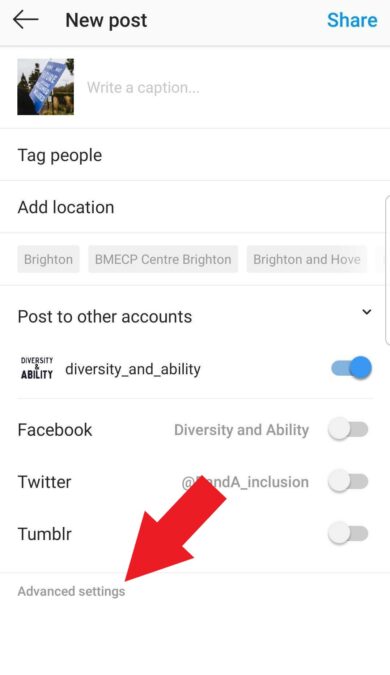This is an image of a social media interface. The upper inch of the image features a light gray background, transitioning to a white background for the remainder of the image. In the top left corner, a prominent black arrow points to the left. Adjacent to this arrow, "New Post" is displayed in bold black font. On the upper right, the word "Share" is written in light blue.

Following this section is the main white area. Directly below the black arrow is a square image frame showing an outdoor scene with trees, grass, and a piece of signage extending from the lower left to the upper right. To the right of this frame, the phrase "Write a caption..." is presented in gray text.

A thin gray border encloses the options below. First, "Tag People" is written in black, followed by another thin gray border. This sequence continues with "Add Location" in black text, bordered similarly.

Three rectangular tabs in light blue with gray lettering are placed horizontally across the interface. Beneath them, a thin line separates the sections with "Post to Other Accounts" written in black. On the right side, a small downward-pointing greater-than sign is visible.

In the section below, on the left side, the text "Diversity & Ability" is displayed, with its stylized form "diversity_and_ability" written to the right. This section includes a toggle switch for activating cross-posting, which is currently toggled on, indicated by a blue light.

Further down on the left, social media platforms Facebook, Twitter, and Tumblr are listed sequentially, each with toggles on the right side, all of which are turned off. In the bottom left corner, "Advanced Settings" is labeled, marked clearly by a large red arrow pointing down specifically at the "S" in "Settings."